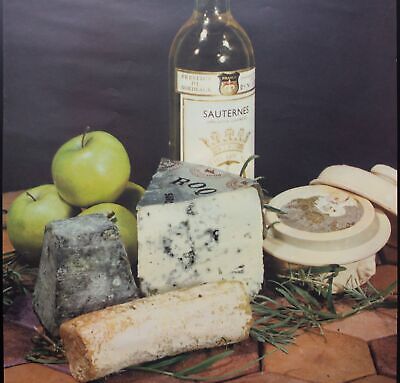This close-up photograph captures an inviting display of gourmet items on a distinct hexagonal wooden tile table, set against a dark blue cloth backdrop. At the forefront, there are three varieties of cheese: a creamy white cylindrical cheese with orange speckles resembling bone marrow, an uncut pyramid-shaped gray cheese, and a slice of moldy blue cheese with blue veining and a gray rind. The table also features a cluster of three green apples, two nestled in a bowl with one balanced on top. A sprig of rosemary lies casually nearby, adding a fresh, herbal element. Adjacent to the cheeses, there's an elegant white ivory stoneware bowl, containing what appears to be a powdery garnish, with a matching lid and spoon inserted within. Dominating the background, a tall bottle of white wine, labeled "Sauternes" in black print beneath a golden crown emblem, adds a touch of sophistication to the scene.